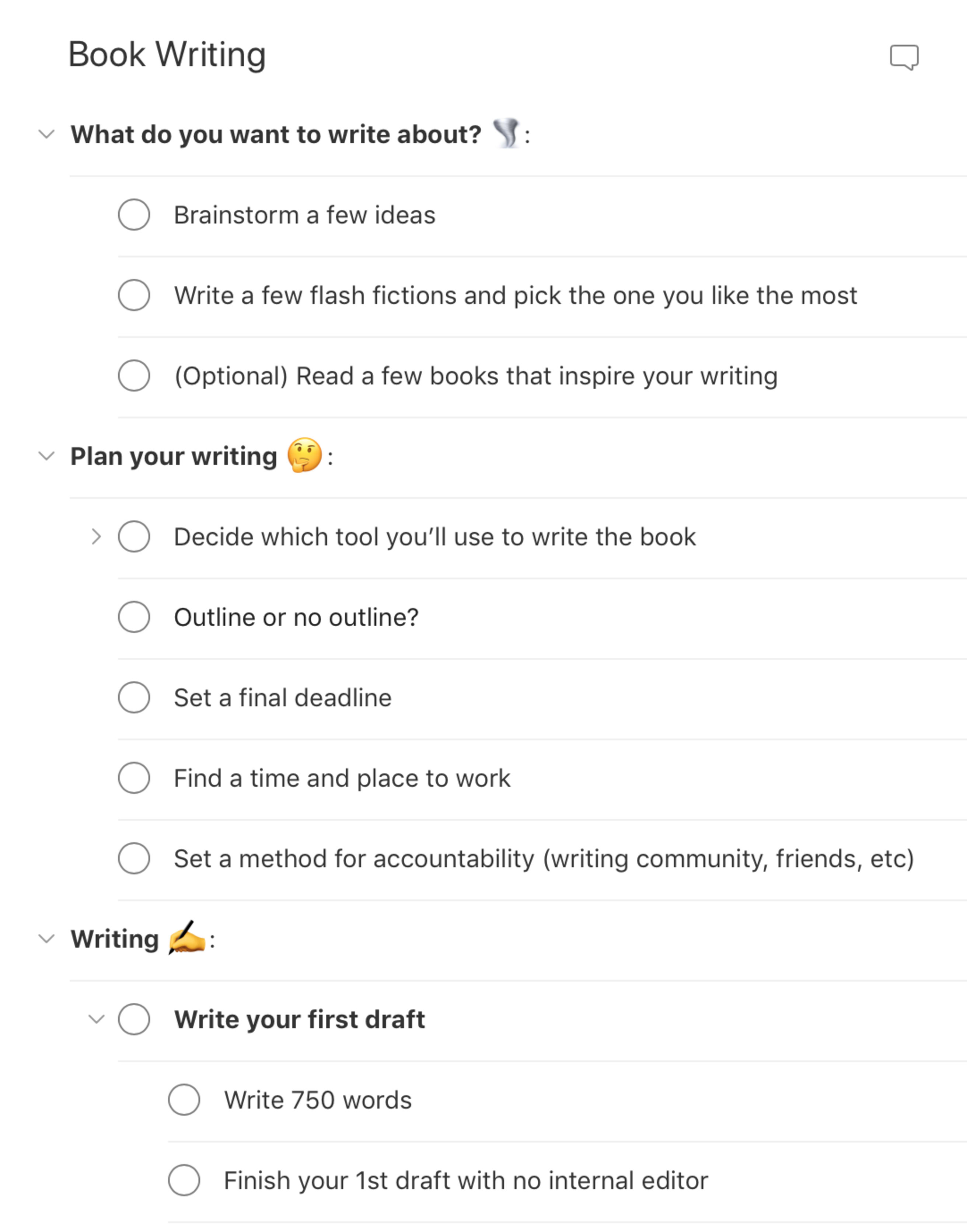The image depicts a detailed webpage focused on guiding users through the book writing process. At the top, the header clearly states "Book Writing," followed by a speech bubble labeled "Chapel." Below this, the webpage is divided into sections with comprehensive steps and tips for writing a book.

1. **Brainstorming**: The first section encourages users to brainstorm ideas with options such as:
   - Decide what you want to write about.
   - Brainstorm a few ideas.
   - Optionally, write a few flash fictions and select your favorite.
   - Read books that inspire your writing.
   
2. **Planning**: The next section, accompanied by a thinking face emoji, provides guidance on planning:
   - Decide which tools you'll use for writing.
   - Choose whether to outline your book or proceed without one.
   - Set a final deadline.
   - Identify a time and place to work consistently.
   - Establish accountability methods through a writing community or friends.

3. **Writing**: The final section focuses on the actual writing process with specific milestones:
   - Write several first drafts.
   - Aim to write at least 750 words consistently.
   - Complete your first draft without internal editing.
   
The page effectively acts as a checklist, where users can mark each step as they progress through the various stages of writing a book. The structured instructions cater to writers of all experience levels, providing a clear and concise roadmap from initial brainstorming to completing a first draft.